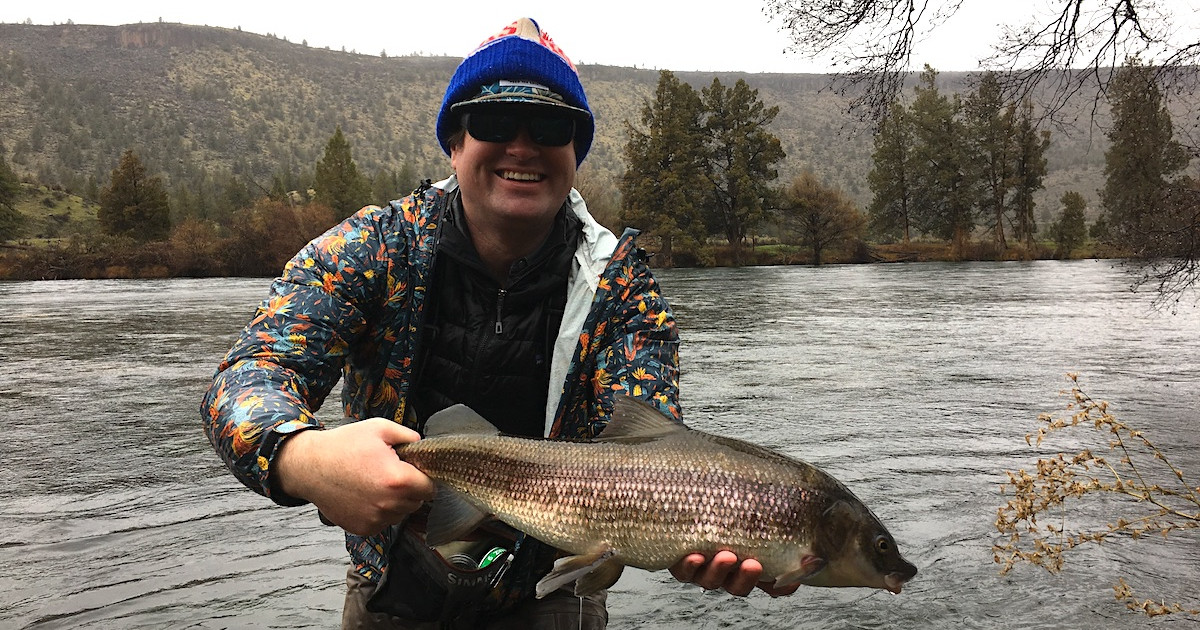In this photo, a man in his 40s stands in the middle of a flowing river, proudly holding a large fish. He grips the fish, which is light brown with a dark, reddish-brown stripe along its middle, by its belly and tail. The fish, possibly a bass, is striking with its dark eyes and closed mouth. The fisherman is dressed warmly in a vibrant, multi-colored puffer jacket adorned with graffiti-like splatters of orange, yellow, and blue over a dark windbreaker. A blue beanie with a hint of red on top covers his head, and he also sports a thick pair of sunglasses. The backdrop features a picturesque and hazy landscape with tall pine and evergreen trees lining the riverbanks. A hilly, forested area extends into the misty horizon, while the sky above appears whitish with a few branches peeking in from the upper right. The water surrounding him has a dark green to brownish hue, adding to the serene and rugged charm of the setting.